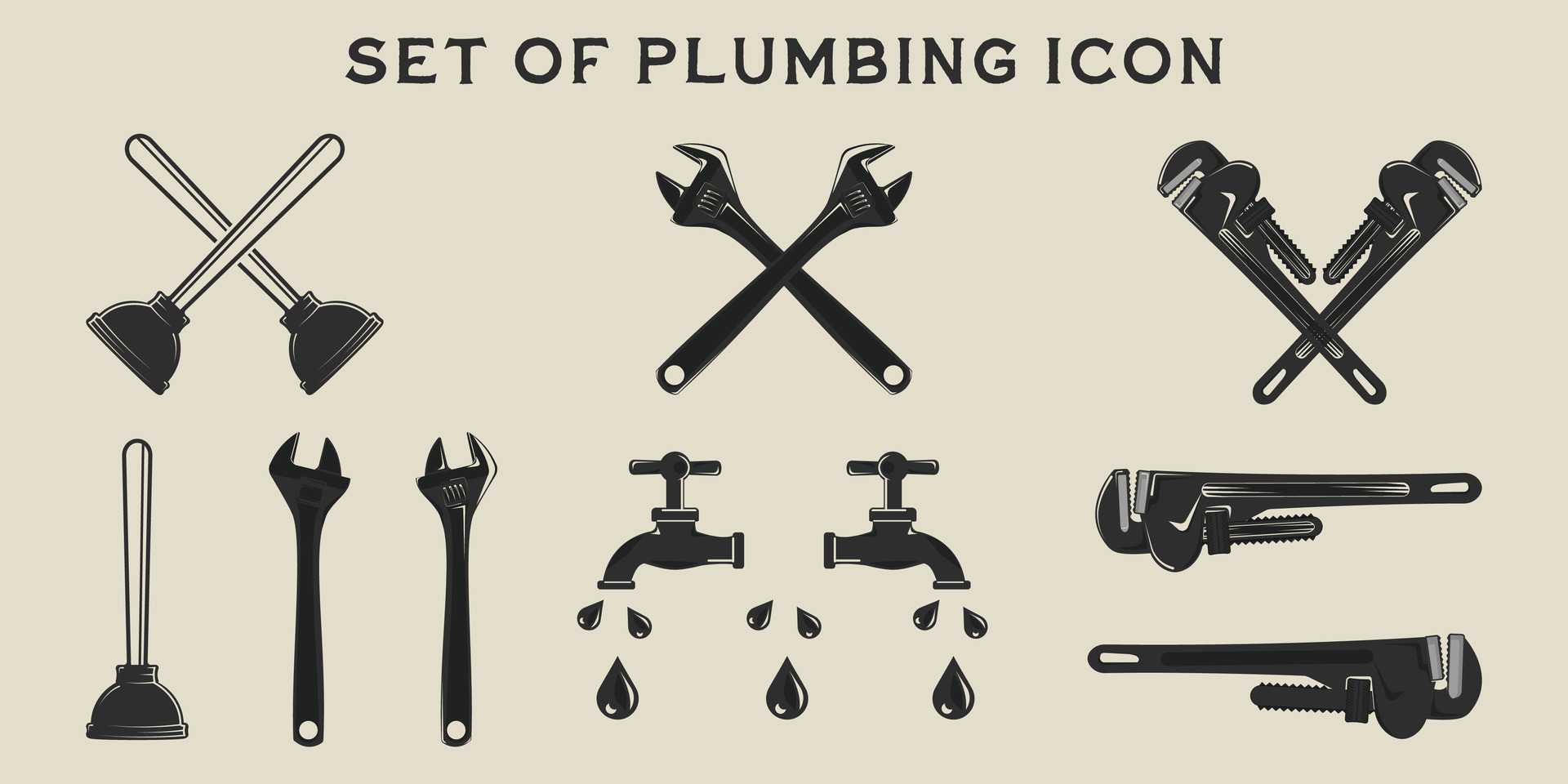The image is a landscape-oriented rectangular illustration featuring a beige background. At the top, in solid, uppercase black font, the caption reads "SET OF PLUMBING ICON." The image consists of two rows of black line-art illustrations of various plumbing tools, presented in a clipart, vector-based style.

In the top row, from left to right, there are three sets of tools: first, two plungers crossing each other to form an 'X'; next, two standard wrenches also crossing in an 'X'; and finally, two specialized wrenches with screws that form an 'X' shape. The bottom row consists of four images: a single upright plunger on the left, followed by two wrenches side by side, then two dripping faucets aligned next to one another, and concluding with two wrenches with screws stacked horizontally. The imagery, devoid of any other text or illustrations, serves as a visual guide to various plumbing instruments.